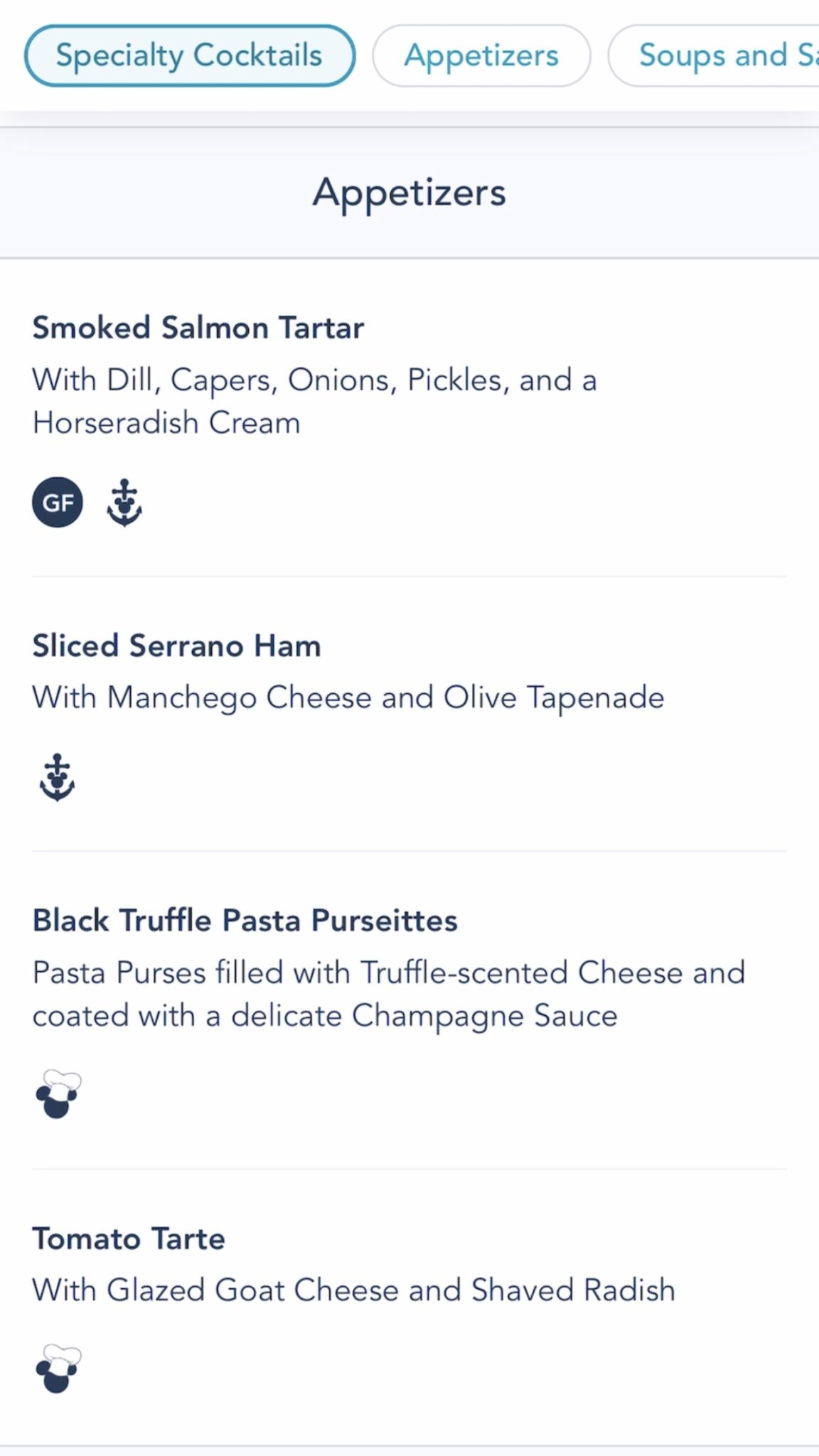The image depicts a section of a restaurant menu on a digital screen. At the very top, there are three discernible tabs, with the currently selected tab titled "Specialty Cocktails" highlighted in light blue, including both the tab's outline and label, which is written in a slightly darker shade of blue. The next tab to the right, labeled "Appetizers," is followed by another tab with the label partially visible, beginning with "Soups and S..."

Beneath these tabs, a light grey banner stretches across the screen, displaying the word "Appetizers" in dark grey text. Below this banner, the menu items are listed, beginning with "Smoked Salmon Tartare," described as being accompanied by dill, capers, onions, pickles, and horseradish cream. Adjacent to this item, a dark grey circle containing the letters "GF" (indicating gluten-free) can be seen, along with a small anchor icon to the right.

The subsequent item, "Sliced Serrano Ham," is paired with manchego cheese and olive tapenade, and is accompanied by a small anchor icon below it. Following this, the menu lists "Black Truffle Pasta Persates," described as pasta parcels filled with a truffle center and cheese, coated with a delicate champagne sauce. Below this item is an icon of a bear's head wearing a chef's hat.

The final item listed is "Tomato Tarte," which features glazed goat cheese and shaved radish, and is also marked with the bear head and chef's hat icon underneath it.